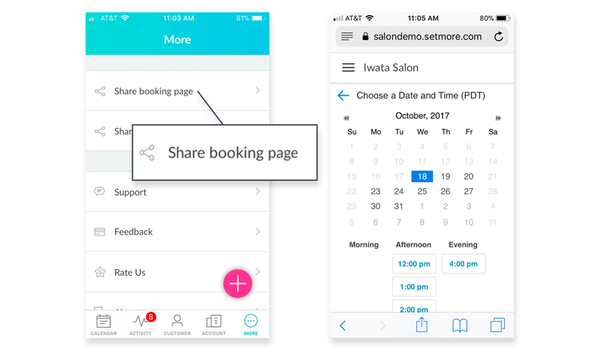The image contains two screenshots, likely from a smartphone, as indicated by their shape and screen size.

In the first screenshot, the phone shows the top bar of an app interface. The status bar displays "AT&T," full Wi-Fi signal, the time as 11:03 a.m., and a battery life of 81%. The top of the screen has a blue header with options like "More" and a highlighted "Share" button. Below the header, the screen shows a magnified section labeled "Share Booking Page" with a list of options including "Share", "Support", "Feedback", and "Rate Us". At the bottom of the app, there are five icons: "Calendar," "Activity" with a red notification badge showing the number eight, "Customer," "Account," and "More." There is also a pink "+" sign.

In the second screenshot, taken two minutes later at 11:05 a.m., the status bar remains the same but the battery percentage has dropped to 80%. The phone is displaying a web page in a private browsing mode. The URL visible is "salon.demo.setmore.com," with the page titled "Iwata Salon." It shows a booking interface for selecting a date and time in October 2017. The current selection is October 18th, with time slots organized into "Morning," "Afternoon," and "Evening." No morning slots are available on this day, but afternoon options at 12, 1, and 2 p.m., and an evening slot at 4 p.m. are displayed, along with a few other available slots throughout the month.